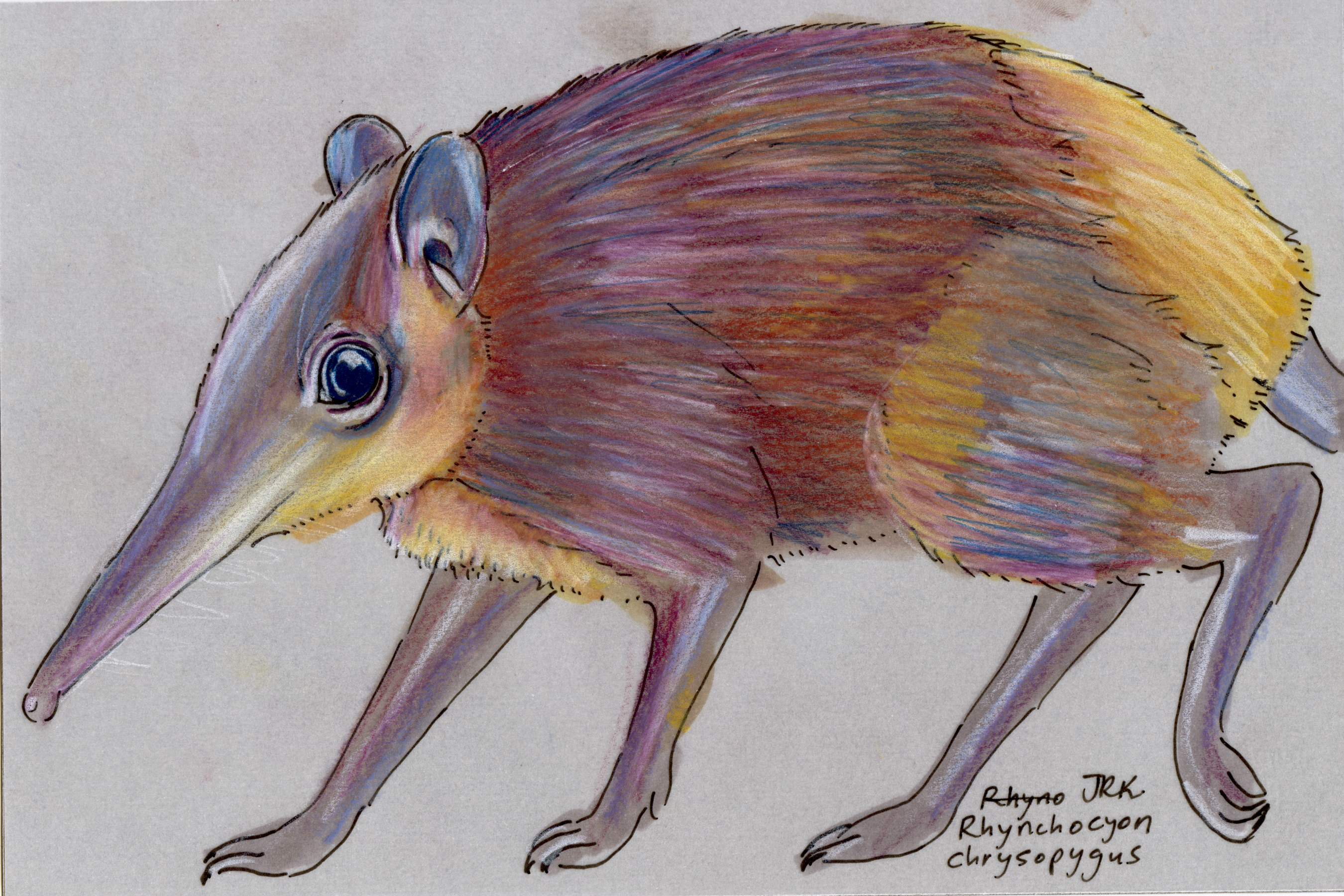The image is a detailed hand-drawn illustration of a unique rodent-like animal, appearing to be created with colored pencils. The creature resembles a cross between a shrew and a mouse, featuring a distinctive long, pointed nose akin to an anteater, but more slender. Its fur is a golden-brown color, similar to that of a hamster, and it has notably long, hairless legs that resemble those of a coyote. The animal is depicted walking towards the left side of the image against a grayish background that mimics paper.

The creature boasts a small face with big eyes, tiny ears, and a rat-like tail. Below the illustration, the Latin name "Rhynchocyon chrysopogus" is inscribed, indicating the species, though the text appears partly scratched out at the beginning. The initials "J-R-K" are also present, presumably identifying the artist. This illustration meticulously combines elements of different animals, resulting in a fascinating and vividly colorful representation.